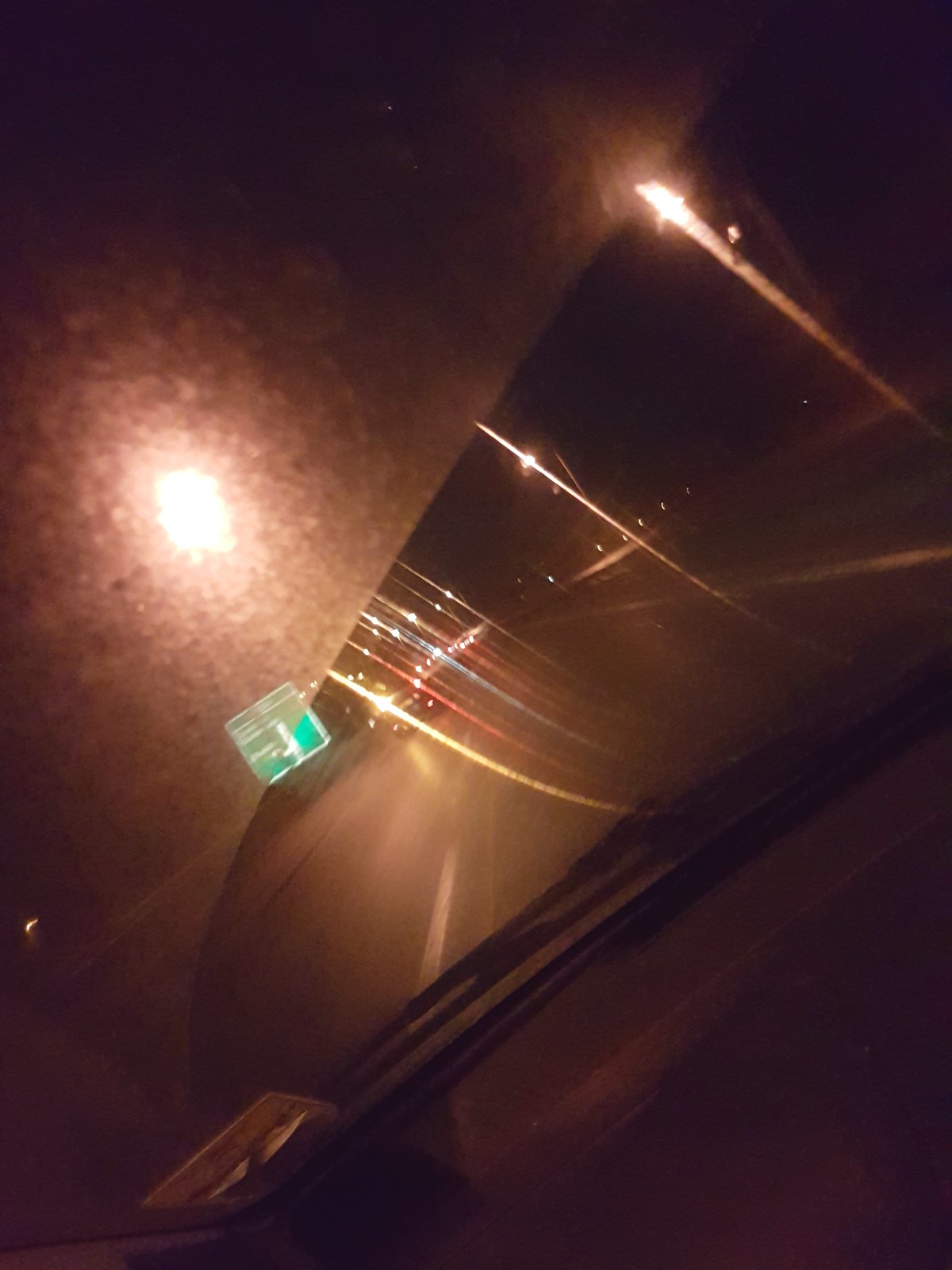A nighttime photograph taken from the driver's side of a moving vehicle, capturing a rainy night scene through a slightly dirty windshield with visible streaks from the wipers. The street lights in the image create a starburst pattern, their reflections casting hues of white, orange, yellow, and red onto the wet, dark pavement. Car taillights and road markings add to the bustling urban environment. A blurry green street sign with white text is visible but unreadable due to the motion and the murky windshield. The image, taken at an angle, emphasizes the dynamic feel of the moment, providing a vivid, albeit chaotic, snapshot of a rainy night drive.